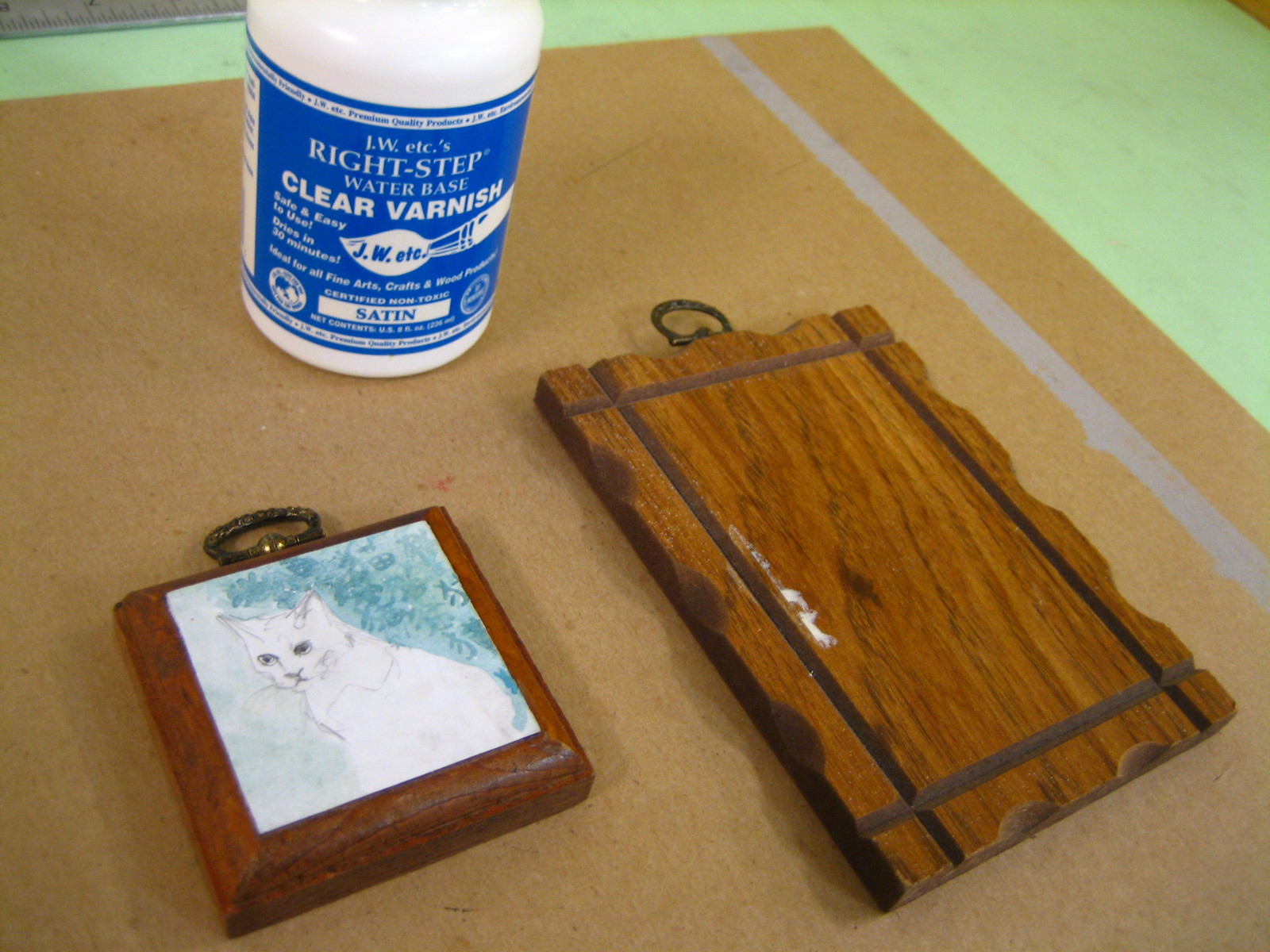The photograph displays three distinct objects arranged on a brown table with a greenish background. At the top, there is a partially visible white bottle with a blue label that reads "Right Step Water-Based Clear Varnish," and it includes text indicating a satin finish and certified non-toxic properties. Below the varnish, towards the center right, is a vertical, rectangular piece of dark brown wood resembling the size and shape of a standard 9.5 x 11-inch sheet of paper. This wood piece features a bronze-colored wall hanger attached to it but no additional markings or images. To the bottom left lies a smaller, square piece of wood adorned with a painted image of a white cat against a gradient background transitioning from light blue to dark blue. The cat is centrally positioned and faces left. These items are arranged in a roughly triangular formation, collectively resting on the table's surface.